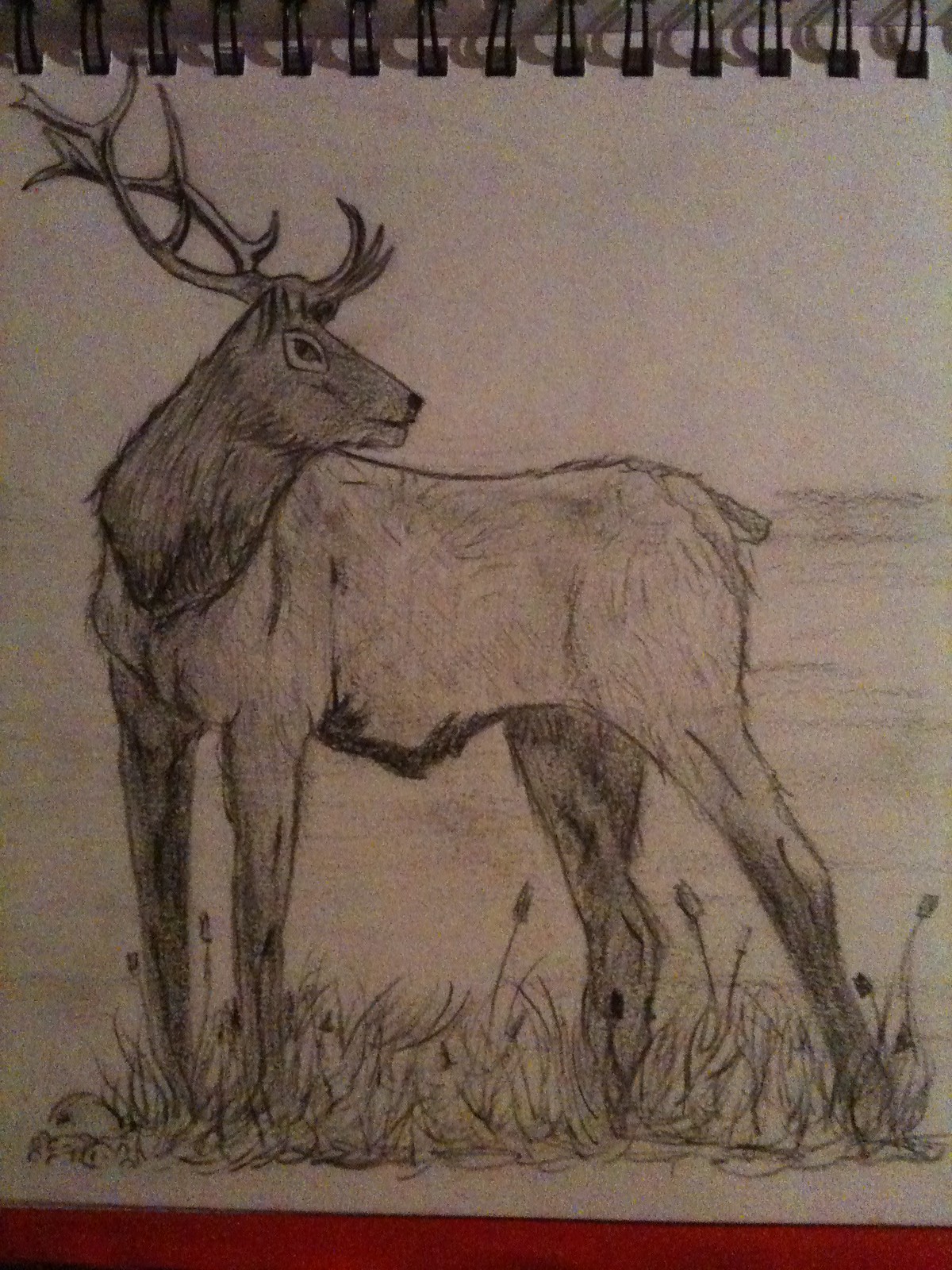This detailed pencil drawing on a spiral-bound sketch pad portrays a male deer with prominent antlers, standing amidst grass and flowers, likely tulips, on a wooden table. Capturing the right profile of the deer’s face, the artist has positioned the animal facing left while looking back towards its tail. The sketch highlights fine details like the white around the deer's eye and subtle hair shading, indicating the light source is from behind. Finished in varying shades of gray pencil on white-gray paper, the sketchbook rests on a red tablecloth visible at the bottom, blending seamlessly into the scene's naturalistic background.